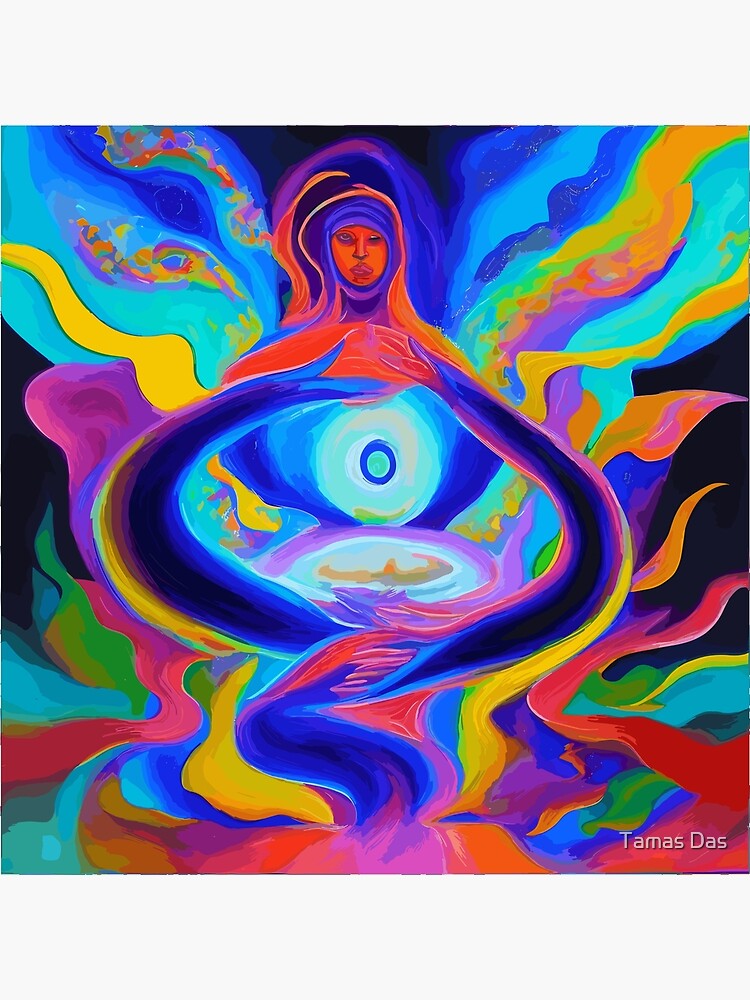This vibrant and abstract digital illustration by Tomas Das features a central figure of a woman whose face appears at the top of the image, partially covered by a blue scarf. The artwork explodes with a myriad of psychedelic colors, including shades of red, orange, blue, green, yellow, purple, and pink, all radiating outward from the woman. A focal point emerges at the center, characterized by an orb with darker blue and green hues surrounded by elements resembling blue and green wings or flames. The lower portion of the image is filled with swirling patterns and colors that contribute to the overall fiery and dynamic feel. The predominantly dark background enhances the vibrancy of the muted yet intense colors, creating a vivid contrast. A watermark at the bottom right-hand corner displays the name "Tomas Das," presumably the artist.